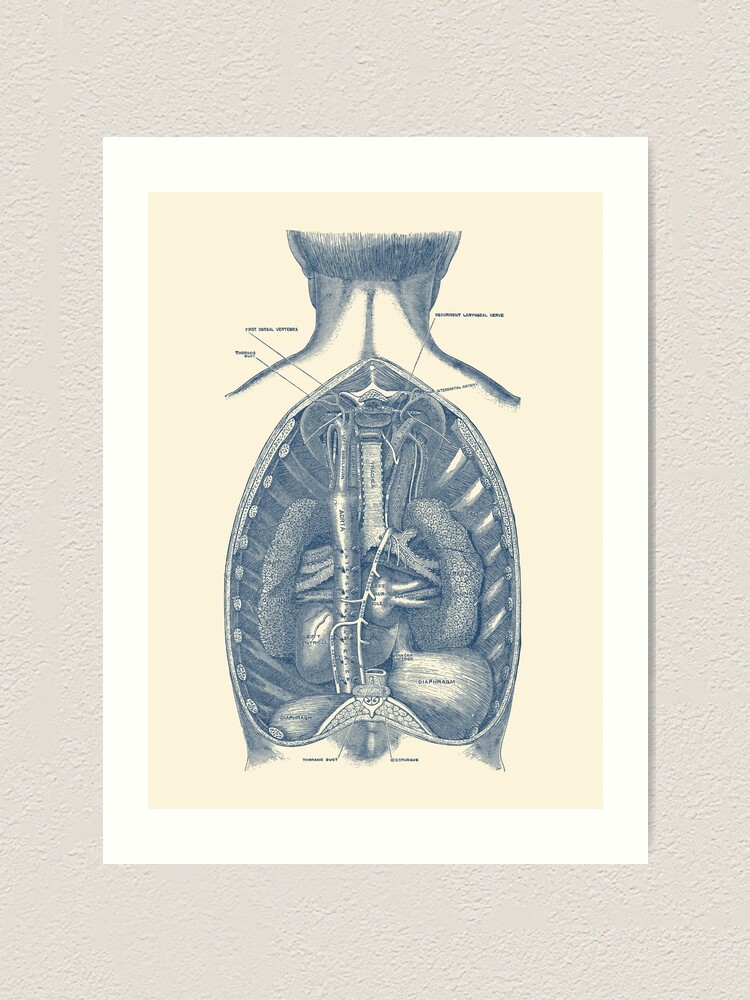The image displays a hand-drawn medical diagram of a human torso, extending from the middle of the head down to the torso, emphasizing detailed anatomical features. The poster, framed in white, is affixed to a wall with a textured surface resembling that of an old apartment or house wall, in a light beige or cream color. The illustration itself features a pale yellow or beige background with a detailed navy bluish-grayish sketch of a man's back, revealing internal organs like the liver, bladder, lungs, and ribcage. Each organ is labeled with small, somewhat illegible text, including three labels near the shoulders and two towards the lower torso. The overall setting suggests a clinical or educational environment, enhanced by the meticulous representation of the human anatomy.